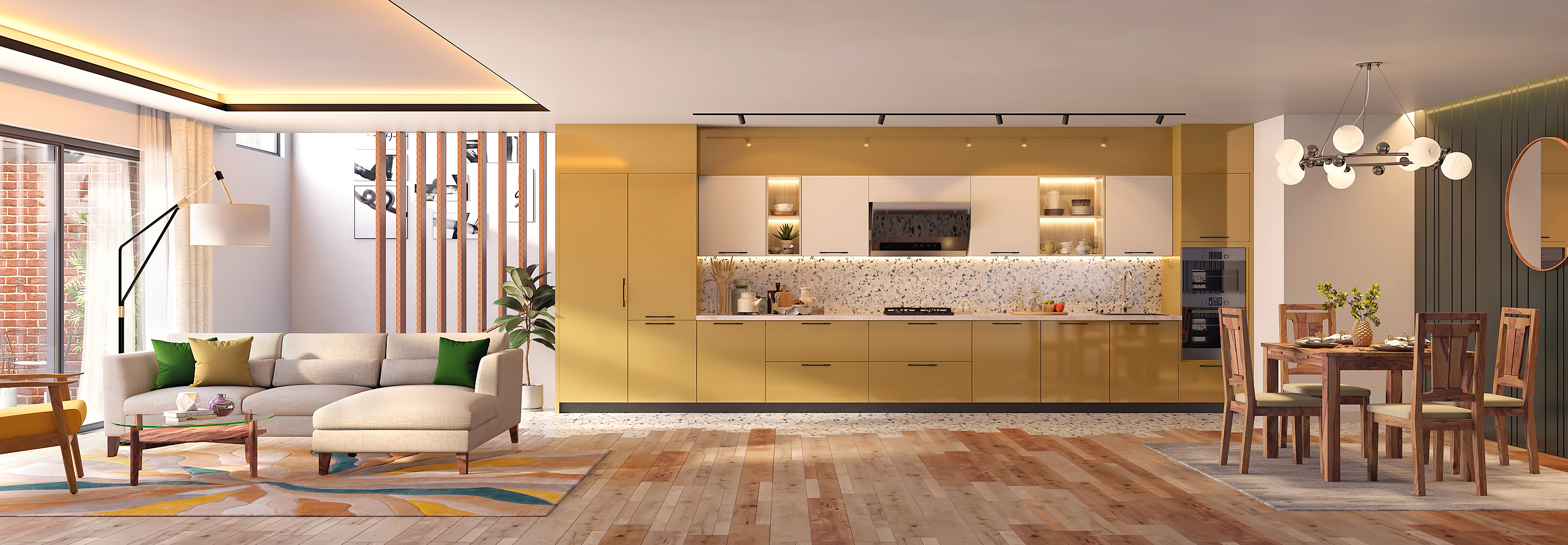The image depicts a detailed 3D render of an apartment interior. On the left side, there is a cozy living room setup with several white-cushioned couches adorned with yellow and green pillows. In front of the couches, there is a small glass coffee table and an additional chair. The living room area is brightly lit by white overhead lights, and notable for a wall featuring a combination of pink and white lights, adding a touch of vibrancy to the setting. To the right of the living room is a dining area that includes a wooden kitchen table set for four people, with plates already laid out. This area is illuminated by a chandelier with spherical lights hanging above the table. The background includes a modern kitchen, characterized by yellow cabinets and various appliances. The kitchen is separated from the dining area by a green wall with a mirror.  The entire apartment features a wooden floor and a rug in the living area, enhancing its cozy ambiance. Furthermore, the back wall of the kitchen area is painted green and includes a sliding glass door that leads to an outdoor patio area enclosed by a brick wall. Overall, the setting exudes a warm and modern aesthetic, with a harmonious blend of colors ranging from beigeish whites to vibrant yellows and greens.